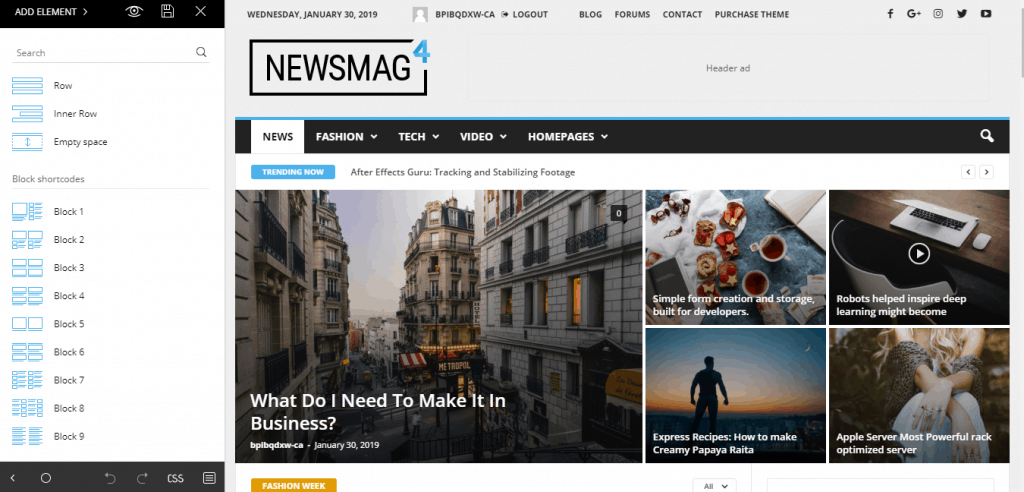The image depicts a web page in the process of being built, featuring several distinct elements and sections. 

In the top-left corner, "Add Element" is prominently displayed in white text. Adjacent to this, there is a small icon, followed by a floppy disk icon for saving, and an 'X' icon to close. Below "Add Element," a menu lists options such as "Search," "Row," "Inner Row," and "Empty Space," as well as "Block Shortcodes" with items labeled from "Block 1" to "Block 9."

Centrally, at the top, a black rectangle with the text "News Mag" is visible, and a number "4" in blue sits at the top-right corner of this rectangle. In the top-right corner of the image, several social media icons are visible, including Facebook, Google Plus, Instagram, Twitter, and YouTube.

The middle section of the image features various square boxes arranged side by side, with one prominent large box in the middle-left area. This large box contains text stating "What Do I Need to Make in Business" and is paired with an image of a cityscape. To the right of this large box, there are four smaller boxes. They display the following texts: "Express Recipes," "Apple Server," "Robot Help Inspire Deep Learning," and "Simple Form Creation."